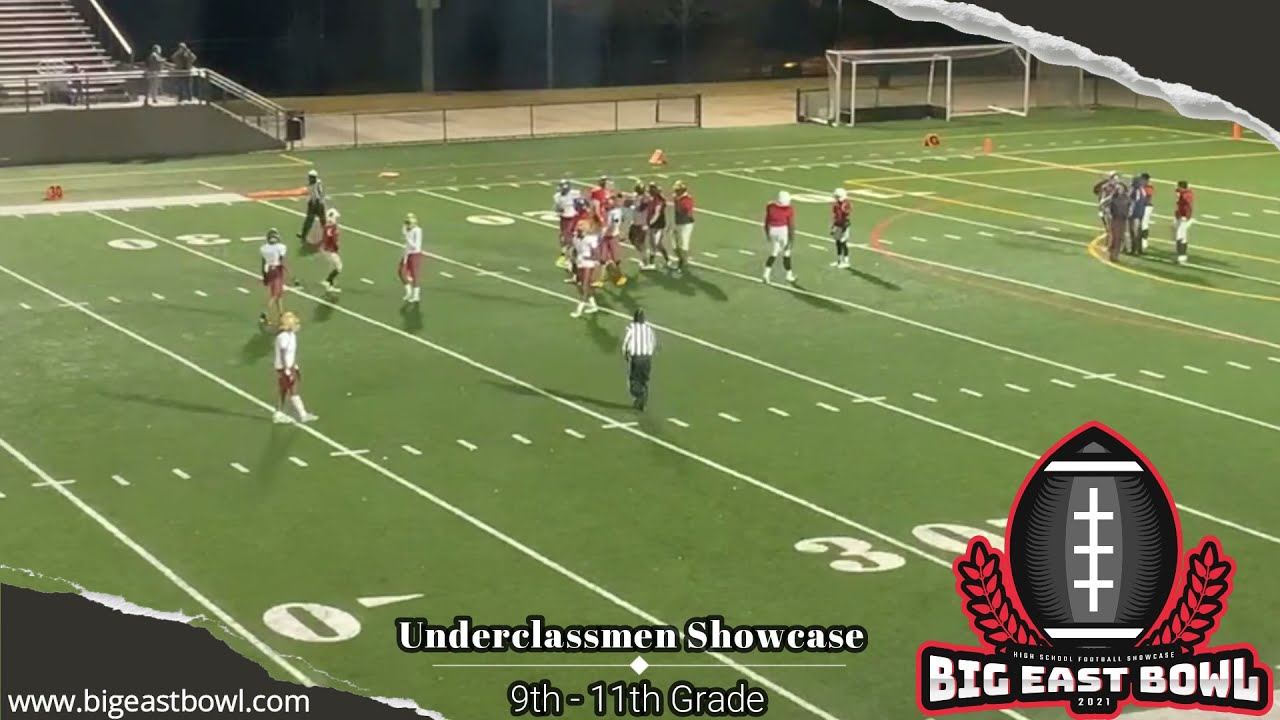The image depicts a high school football game during the Big East Bowl 2021 Underclassmen Showcase, meant for 9th to 11th graders. In the foreground, a mix of football players and referees are positioned primarily around the 30-yard line, which is visible both near the bottom right corner and in the upper left corner. The scene spans approximately 30 yards of the field, capturing the dynamic movement of the players and referees in various positions. The playing field is lush green with crisp white yard lines, enhancing the vividness of the players' red, white, and yellow uniforms contrasted against the black and white attire of the referees. 

In the bottom right corner, there's an emblem featuring a black football with white laces, outlined in red with red grain imitations around the edge, which prominently reads "Underclassmen Showcase" in the center and "Big East Bowl 2021" underneath, followed by "9th-11th grade." The website "www.bigeastbowl.com" is printed in black in the bottom left corner. 

In the background, the mostly empty stadium seats are discernible, with two individuals standing by a barrier on the stairs. On the upper right, tucked away soccer goals are visible, and a barrier with a black metal bar and an open gate runs along the top of the image. This setting appears to be a screenshot from a live-streamed event, capturing the essence and energy of a high school sports showcase.